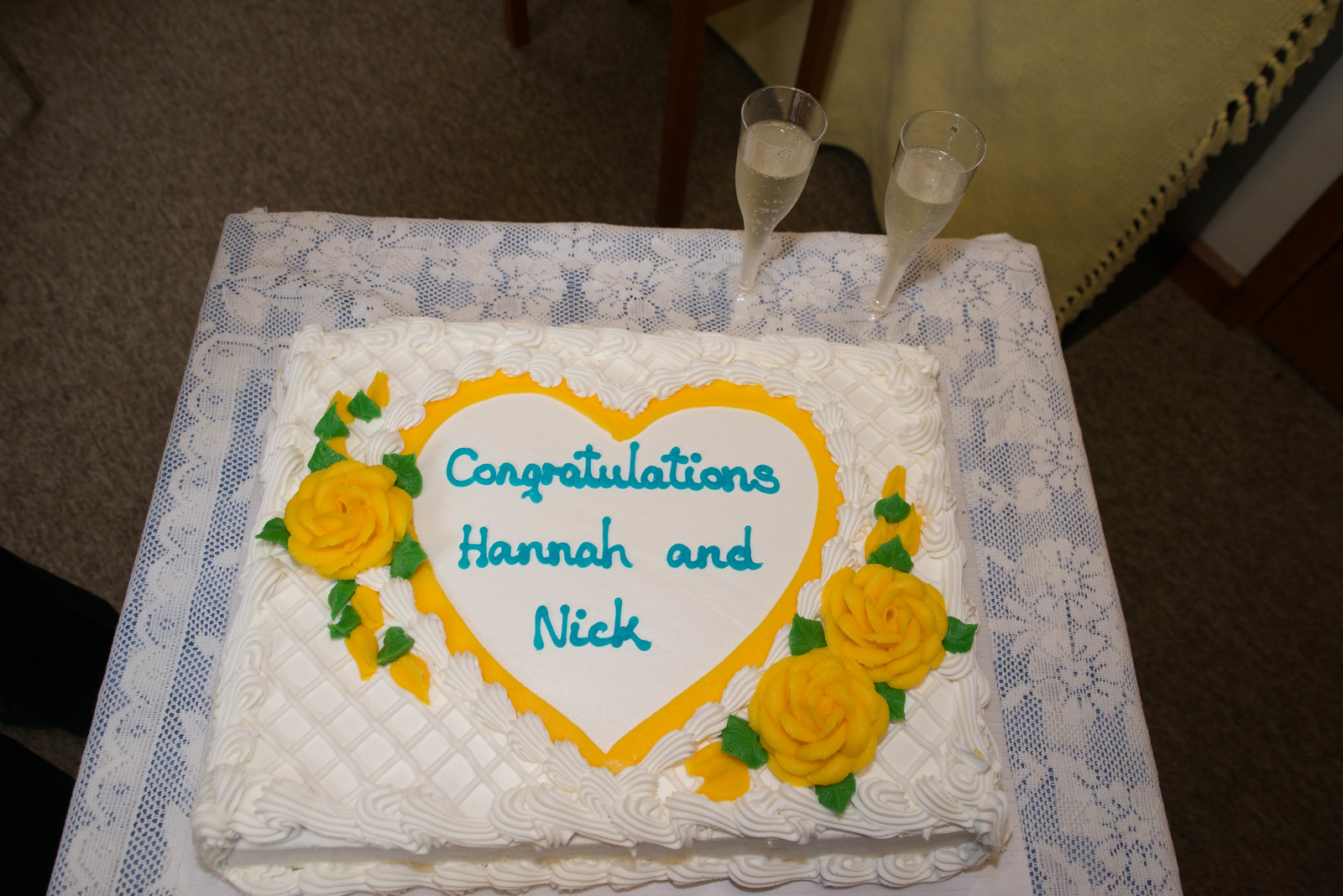This full-color indoor photograph captures a celebration scene centered around a beautifully decorated cake. The cake, enrobed in white frosting, features a yellow heart in the middle, inscribed in blue cursive with “Congratulations, Hannah and Nick.” The cake is adorned with two yellow frosting flowers in the lower right corner and one in the upper left corner, complete with green leaf accents. It sits on a small card table draped with a white lace tablecloth, which displays flower motifs. Positioned on a tan shag carpet, the scene also includes two filled champagne flutes at the top right corner of the table. Details like a snippet of spiral notebook paper in the upper right corner and a glimpse of brown curtains further frame this indoor festivity, making it clear that this heartfelt celebration is taking place in a cozy home setting.